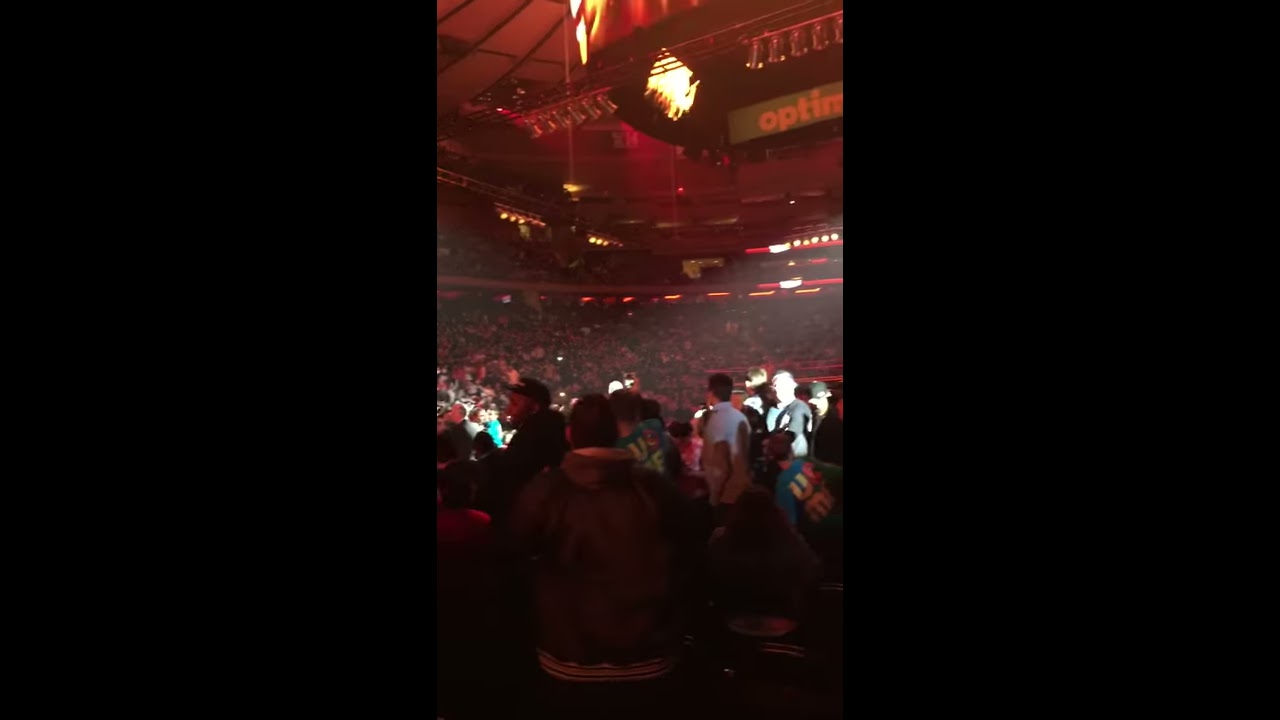The image portrays a large, crowded arena that suggests a bustling event, possibly a concert or a sporting event involving a boxing ring, as indicated by visible ropes in the middle right of the photo. The photograph is part of a three-panel layout with black panels flanking the image. Shot from the back of the auditorium, the picture captures a densely packed crowd both in the foreground and middle ground, with many attendees facing away from the camera. The upper levels are dimly lit, making it hard to discern details, but they appear to be filled with people as well. Notably, there is a bright light emanating from the right side, casting intense illumination and causing some individuals to face it, obscuring their facial features. A partial banner displaying the word 'OPTIM' is visible, and numerous lights are mounted on a metal beam at the top of the arena, contributing to the overall bright ambiance.